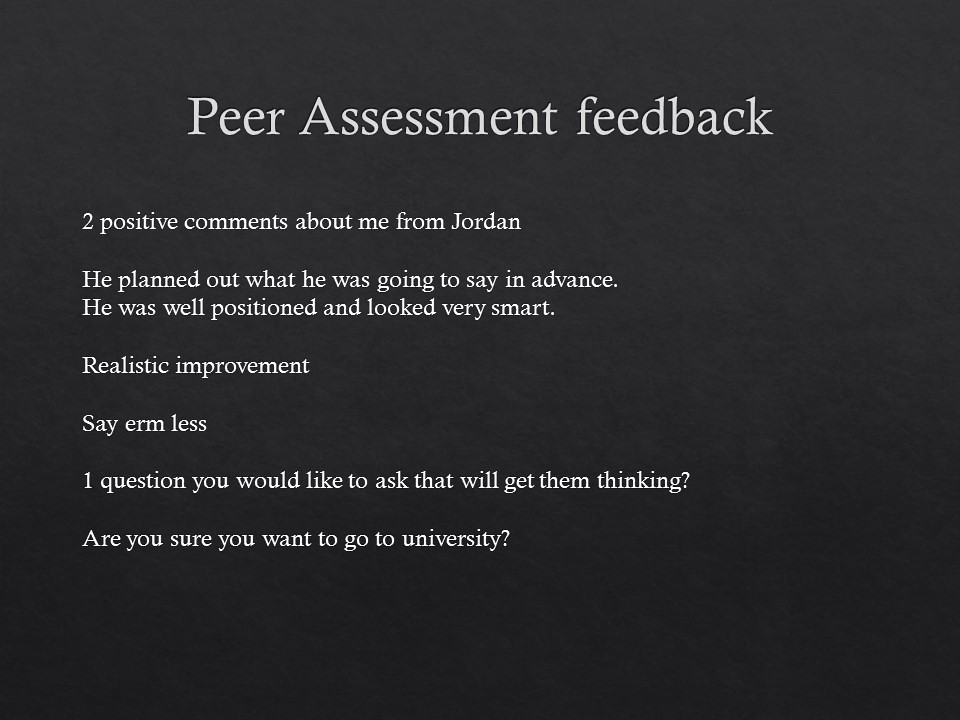The image is a screenshot of a digitally created document with a black, textured background. The document is headed with large white text reading "Peer Assessment Feedback." Below this title, in smaller white text, are several structured points. The first section, titled "Two positive comments about me from Jordan," includes: "He planned out what he was going to say in advance. He was well-positioned and looked very smart." The next section, labeled "Realistic improvement," advises: "Say 'erm' less." Following this is a prompt: "One question you would like to ask that will get them thinking," with a sample question: "Are you sure you want to go to university?" The text-only layout of this document, almost flashcard-like in style, appears to be an academic peer review, potentially for educational settings such as high school or college. The feedback focuses on constructive criticism and thoughtful questioning.